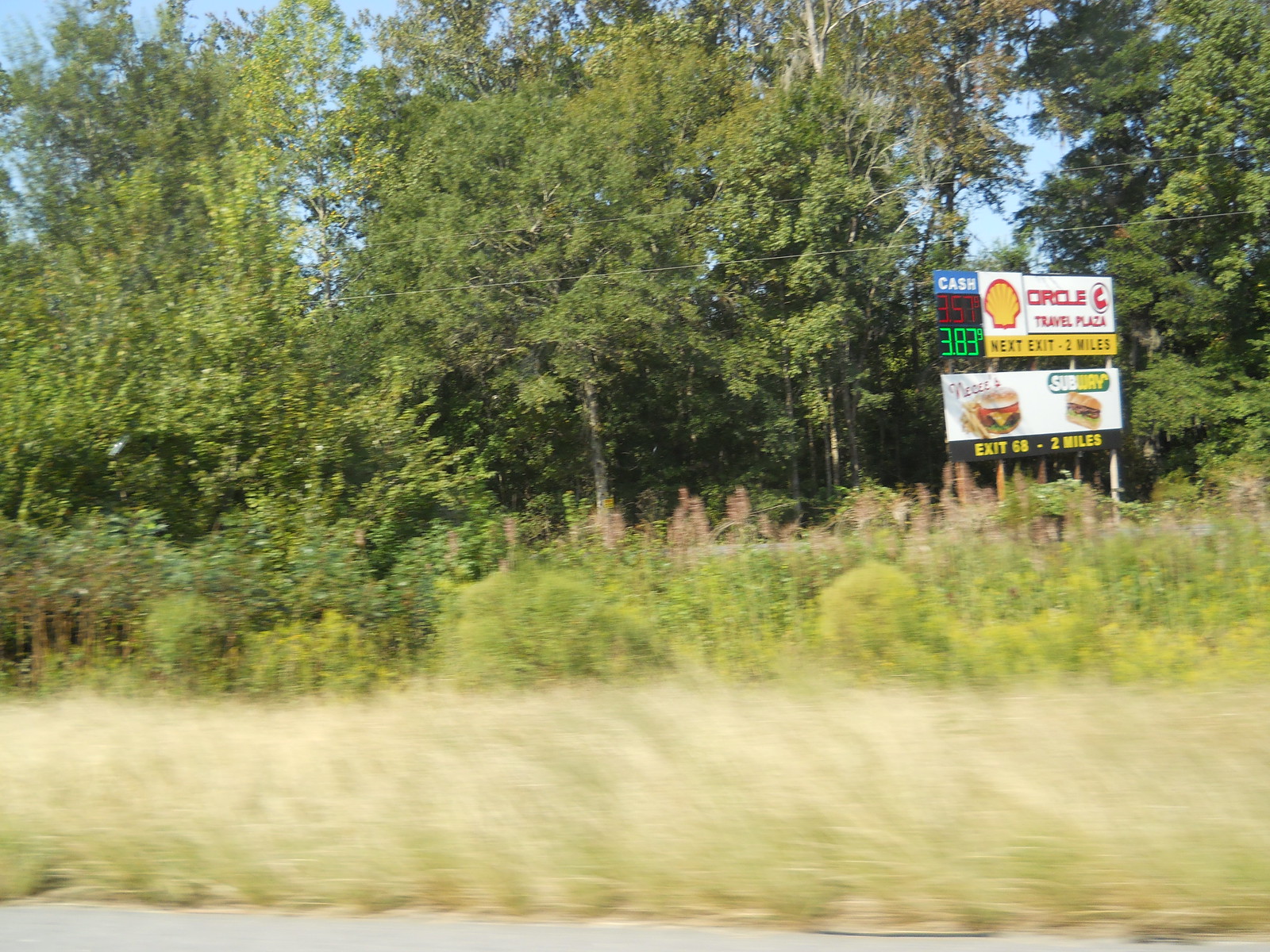This daytime photograph showcases a landscape foregrounded by tall, overgrown grass of a pale green hue. The middle ground features additional grass and bushes, displaying a spectrum of greens from dark to yellowish and pale shades. In the background, a series of billboards rise above the brush, providing various advertisements and information. 

On one side, a striking blue billboard with white font promotes "Cache," accompanied by a digital display presenting gas prices of $3.57 and $3.83. Adjacent to this, there's a prominent Shell gas station logo in yellow and red, followed by a red and white sign for "Circle C Travel Plaza." Below this, another billboard advertises Subway, displaying the iconic white, green, and yellow logo along with an appetizing image of a Subway sandwich on a white background.

On the opposite side, another billboard slightly obscured by distance features an eatery advertising a burger and fries, accompanied by the text "Exit 68, 2 miles" in bold yellow letters. The mixture of natural elements and commercial signage creates a vivid snapshot of a roadside area bustling with visual interest and information.